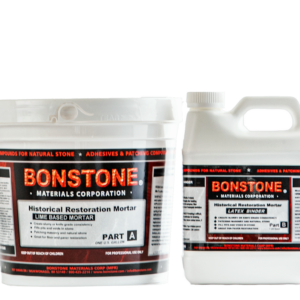Against a white backdrop, the image showcases two white plastic containers used for historical restoration mortar, produced by Bondstone Materials Corporation. The container on the left is a large bucket equipped with a screw cap lid and handle, designed for pouring. On the right is a sizable jug, likely a 5-gallon refill bottle. Both containers are adorned with detailed labels featuring the Bondstone logo in orange text on a black background, with "Materials Corporation" written in white underneath. The labels, affixed to the front and fully encircling the containers, also include the product description: "Historical Restoration Mortar, Lime Based Mortar." The bucket is labeled as Part A, while the jug is marked as Part B, indicating that they complement each other in use. Additionally, the labels feature circled text mentioning "Adhesives" and "Natural Stone," further emphasizing the product's application in restoration work.